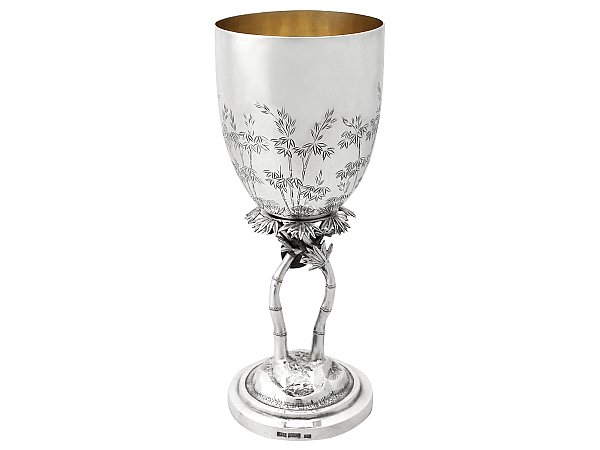The image depicts a detailed and intricately designed chalice, primarily metallic in appearance. The base is a whitish silver platform, featuring some black writing that is illegible. From this base, two bars resembling tree trunks rise and culminate into palm trees, which act as the stand for the cup. The main cup is adorned with intricate engravings of palm trees and leafy branches, continuing the arboreal theme. The exterior of the cup has a shiny, whitish silver hue, while the interior contrasts beautifully with a warm gold color, possibly of copper or brass. The entire piece is set against a plain white background, highlighting its detailed craftsmanship and striking metallic hues. The principal colors in the image are black, gold, silver, and white.